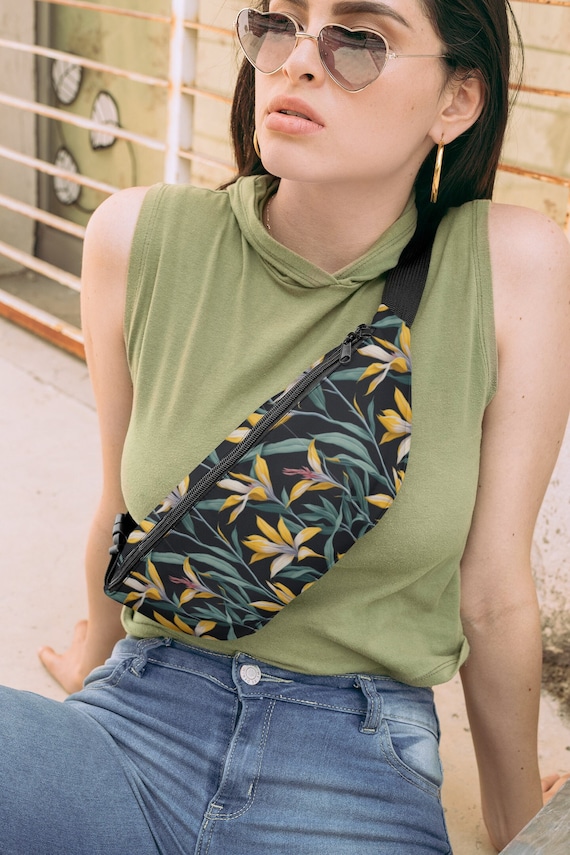The image captures a young brunette woman, likely in her early 20s, seated on what appears to be a sidewalk or concrete surface. She exudes a trendy fashion sense, wearing heart-shaped sunglasses and gold hoop earrings. Her outfit consists of a lime green tank top with an army green hoodie, complemented by faded blue denim jeans. A floral-patterned fanny pack—adorned with yellow and white flowers, as well as green leaves—is stylishly draped across her chest from her right shoulder to her left waist. She is leaning back on both of her arms, gazing away from the camera, presenting a relaxed yet fashionable pose.